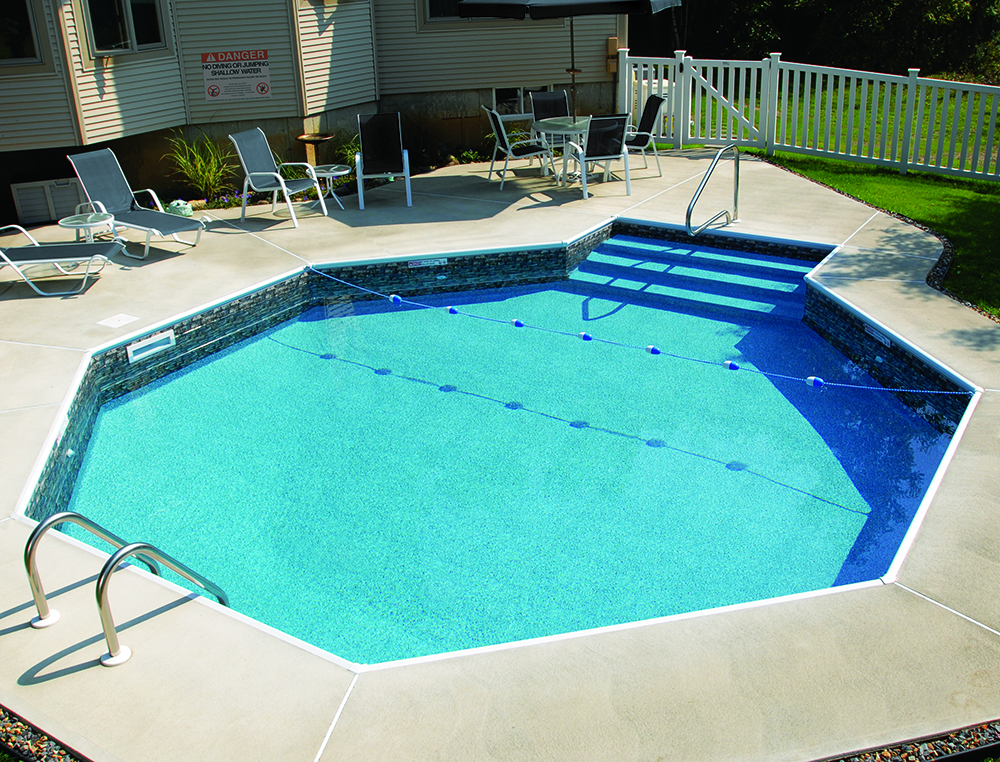This detailed image depicts a geometric swimming pool with a hexagonal/octagonal shape featuring three steps leading into the bright turquoise blue water. The pool is equipped with chrome-colored railings for support on either side. A floating string stretches across the surface of the water, adding to the pool's safety measures. Surrounding the pool is a dull gray, cement-paved area adorned with outdoor furniture, including chairs positioned on the top left side of the image. In the top right corner, a classic, white-painted wooden fence encloses part of the area while a patch of grass is visible on the right side. To the left, there's a building with white-striped walls, closed windows, and a sign, indicative of a home exterior setting. This setting offers a serene and functional outdoor space, perfect for relaxation and enjoyment.